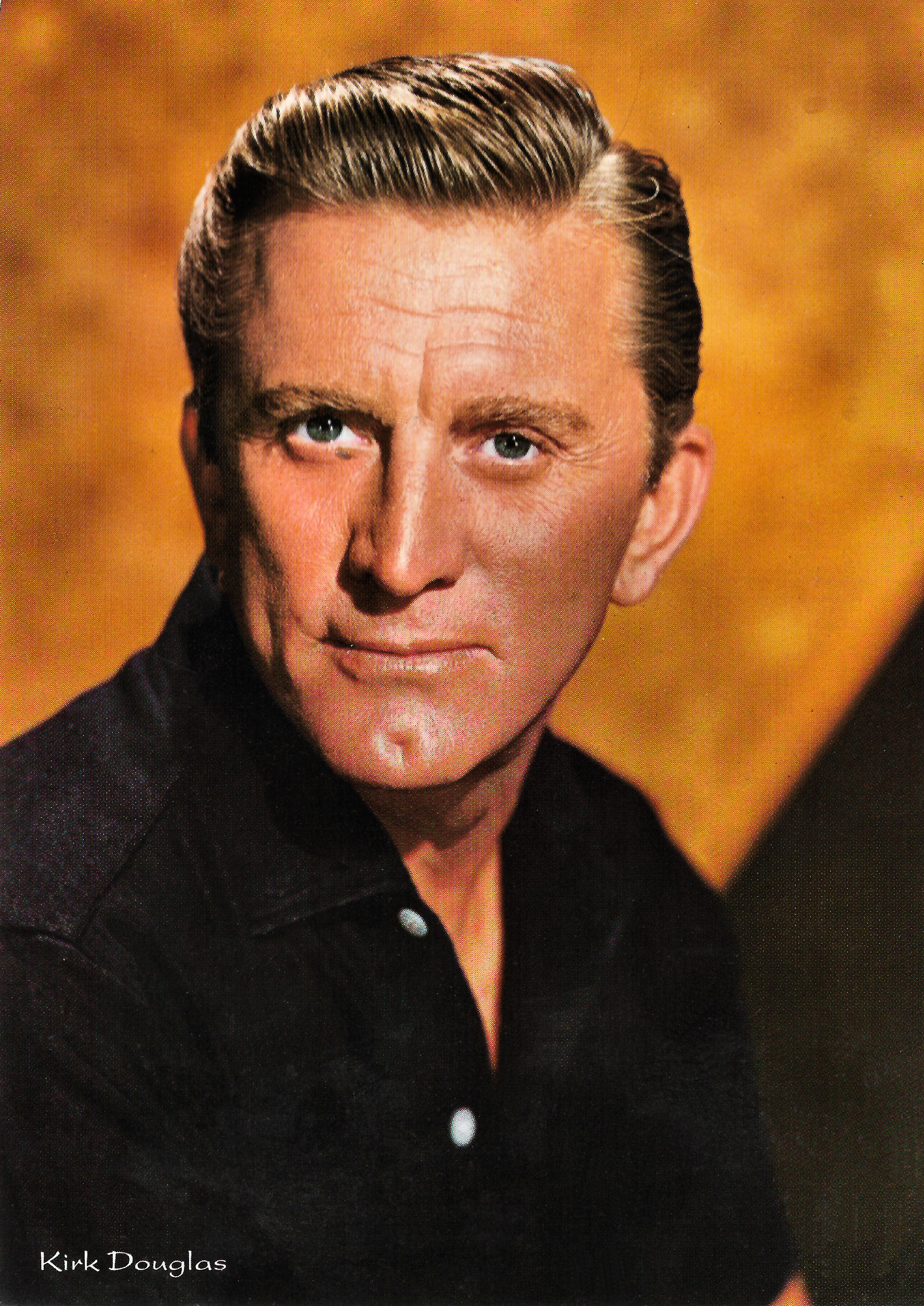This close-up portrait photograph features the iconic actor Kirk Douglas, his name displayed in small white letters at the bottom left corner. Douglas's intense gaze is directed straight at the camera, accentuating his piercing blue-green eyes. His meticulously styled, slicked-back light blonde hair and matching eyebrows frame his rugged face, highlighted by a distinct chin dimple. He is dressed in a black button-up shirt with a collar, one button left undone. The background is a solid, blurry gold color, with a patch of black in the bottom right corner, drawing all attention to Douglas's compelling expression and presence.